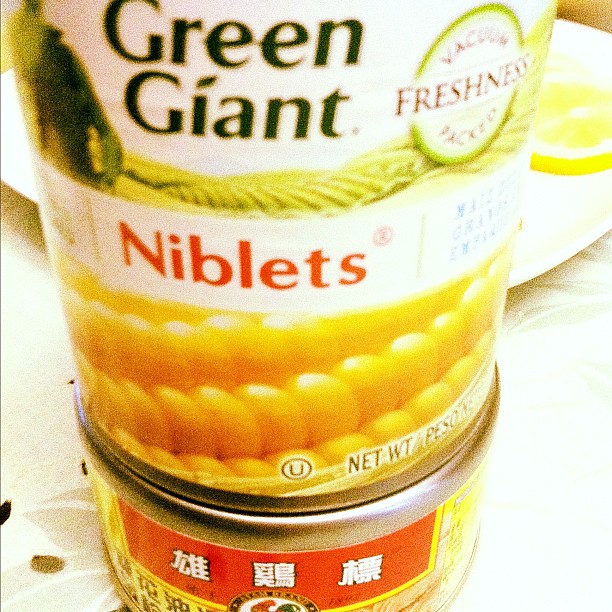The image depicts two aluminum cans stacked on top of each other, set on what appears to be a table adorned with a flowery tablecloth. In the background, there is a white paper tray with a sliced lemon situated in the upper right corner.

The top can prominently features English writing with the brand name "Green Giant" displayed next to an image of a green giant on its left side. Below the brand name are rolling hills, emphasizing the natural freshness of the product. To the right, there is a green circle with the word "freshness" in all capital letters breaking the circle's boundary, flanked by horizontal lines. Above this, the word "vacuum" is curved, and at the bottom, it states "packed," making the full phrase "vacuum freshness packed." In the middle of the can, a white band showcases the word "Niblets" in bold red letters, with additional text to the right. The bottom third of this can displays an image of corn on the cob and includes an emblem - a circled "U", along with weight details indicated by "Net WT."

The bottom can is shorter and features writing that appears to be in either Chinese, Japanese, or Korean. It has a label that might resemble a piece of paper wrapped around the can. The label includes a red rectangle at the top, a circular seal with English text that is somewhat unreadable, and an interior white circle with a red and green design. The label also contains yellow sections with black writing.

The detailed visual elements and the bilingual labels on the cans suggest a blend of familiarity and exoticism, catering to multiple markets.